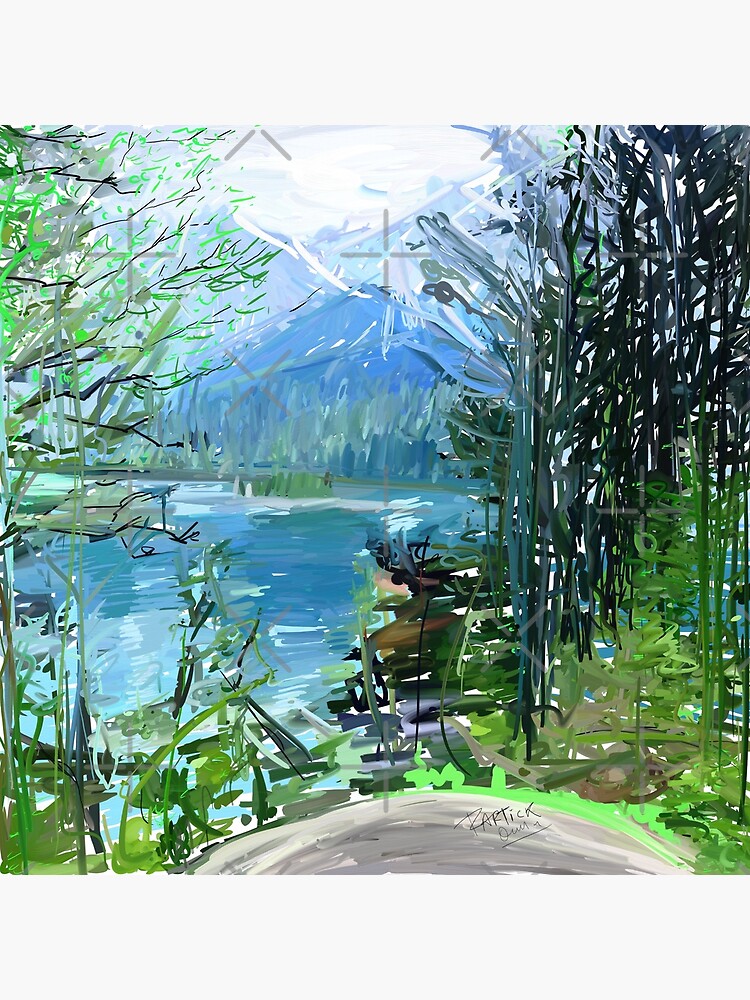This image showcases a detailed landscape painting of a natural scene, likely created with acrylics. The focal point is a serene blue river or lake, adorned with white reflections or markings. Surrounding the water, various shades of green vegetation, including shrubs and long plants, are visible. On the left-hand side, there are trees with thin brown branches and green leaves, whereas on the right, the trees are darker, with trunks appearing in shades of dark blue, black, and even lighter blue.

In the background, the painting reveals triangular bluish mountains, indicative of distance and elevation, with some peaks possibly covered in snow or appearing as clean stone. Above the mountains, a white cloud floats in a sky painted in a light blue hue, adding depth to the scene. The painting captures the view from a hiking trail, offering an elevated perspective over the lake and forest below.

At the bottom of the image, a gray section contains the artist's signature, "Patrick," although this detail was noted by some observers and not by others. The painting also features several gray X's and plus signs scattered throughout. No human figures are present, emphasizing the untouched beauty of the natural environment.